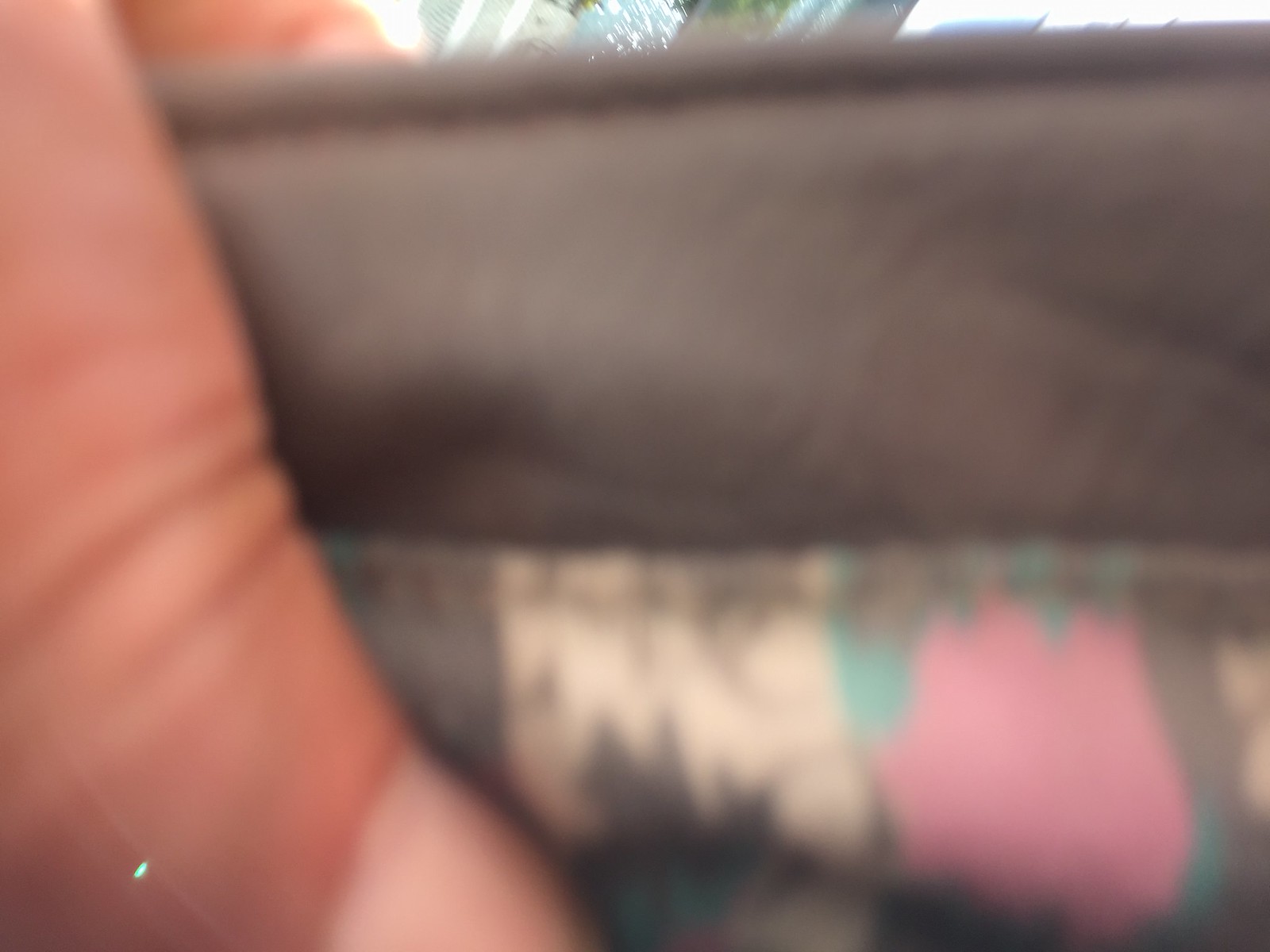A close-up image depicts a right hand holding what appears to be a wallet made of dark brown leather. The wallet is crafted from fabric and features a distinctive Aztec print design in shades of beige, dark brown, teal, and pink on the lower two-thirds of its surface. The person's thumbnail, part of a dark tan hand, is visible at the top of the wallet, adding a human touch to the intricately designed accessory.